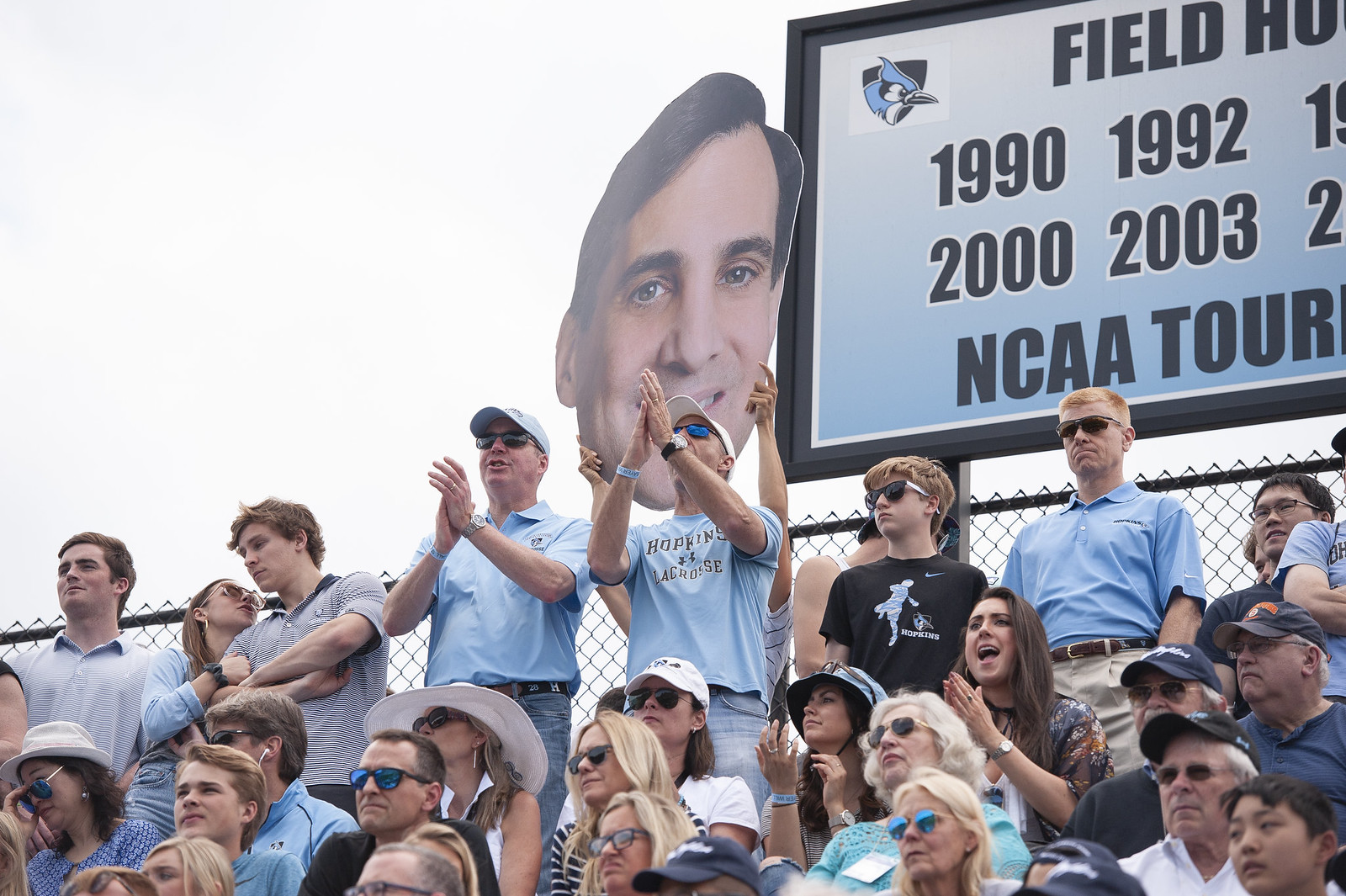The image depicts a lively crowd at an outdoor sporting event, likely an NCAA baseball tournament, given the various references to "NCAA" and the years 1990, 1992, 2000, and 2003 mentioned on a partially visible sign. The weather appears overcast, with the sky a uniform white shade. Many spectators are cheering in the bleachers, wearing light blue shirts, some of which bear the name "Hopkins." A notable feature is a blue and white board in the background, outlined in black. This board bears the partially obscured text including "FIELD" and "NCAA Tour," along with a depiction of a bird in the top left corner. Several fans wear sunglasses, warding off the bright light. 

Among them, a striking element is a sign held up featuring a man's smiling face, possibly a player or a figure the crowd is cheering for. The details showcase an exuberant atmosphere typical of a collegiate sports gathering, with individuals energetically participating in the event.